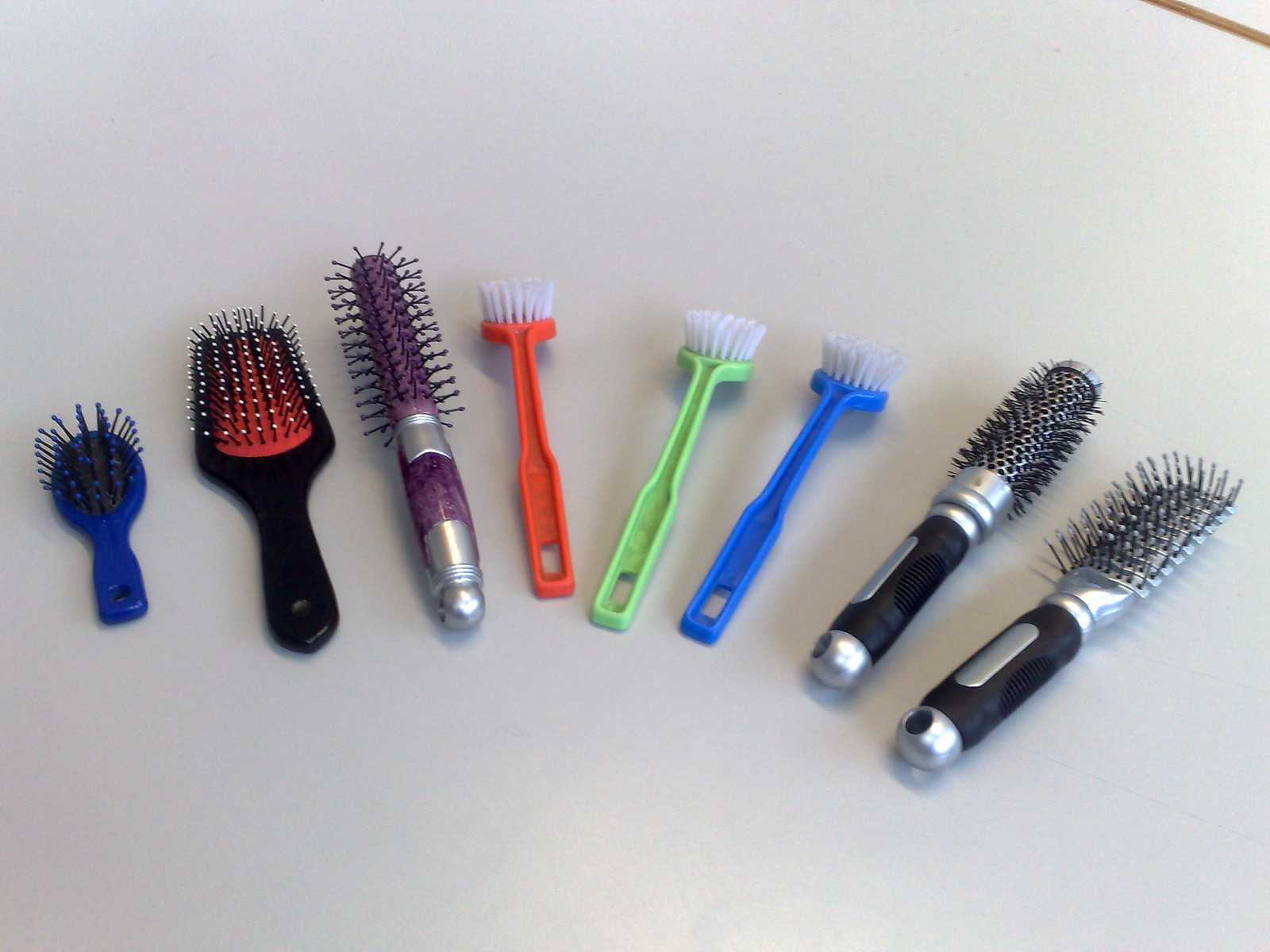The digital photograph captures a collection of nine brushes laid out in an arch-like pattern on a completely white background, with the exception of a green piece of string trailing from the upper portion of the image to the upper right corner. Among the brushes are five hair brushes and three scrub brushes. 

Starting from the left, the first hair brush is a small, dark blue brush with black prongs and blue-tipped ends. It is followed by a black brush with a red base and black prongs featuring silver tips. Next is a silver and purple, round hair brush with black bristles that have purple ball ends. 

The central part of the photo features three colorful scrub brushes with round heads and white bristles. These scrub brushes are red, green, and blue.

To the right of the scrub brushes, there is a black, round-headed hair brush with black prongs. Alongside it is an almost identical brush, but more oblong in shape, also with black prongs and a similar black and silver design.

The brushes are predominantly made of plastic, and most feature plastic bristles, with at least one having fine nylon bristles. The laid-out arrangement and the vibrant colors of the brushes create an appealing visual contrast against the stark white background.